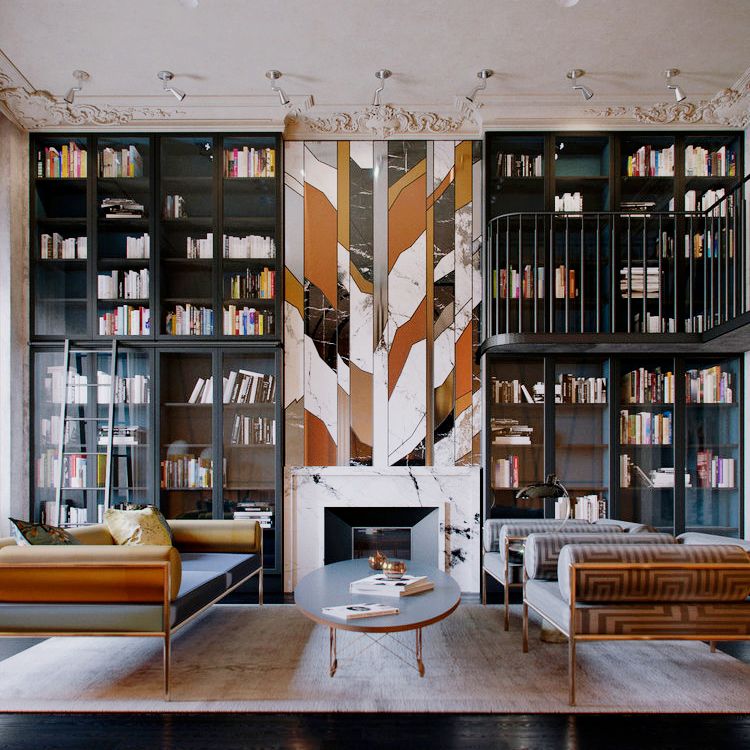This full-color photograph, taken indoors with a mix of natural and artificial light, depicts a vertically rectangular image of an ornate private home library. The bottom border is marked by a black line, representing the floor. Dominating the background are tall bookshelves, partially filled with books and featuring sections enclosed by glass casings. At the center left stands a silver ladder, enabling access to the upper shelves. 

A grand white marble fireplace, adorned with an intricate mosaic of orange, black, and brown hues above it, is flanked by the bookshelves. To the right, a railed walkway serves as an alternative to the ladder for reaching higher shelves. 

The room is furnished with a long, blue couch with gold armrests, and two matching easy chairs, each boasting low backs and overstuffed armrests. These pieces are arranged around a central coffee table and situated on a rug before the fireplace, creating a cozy sitting area amidst the literary surroundings.